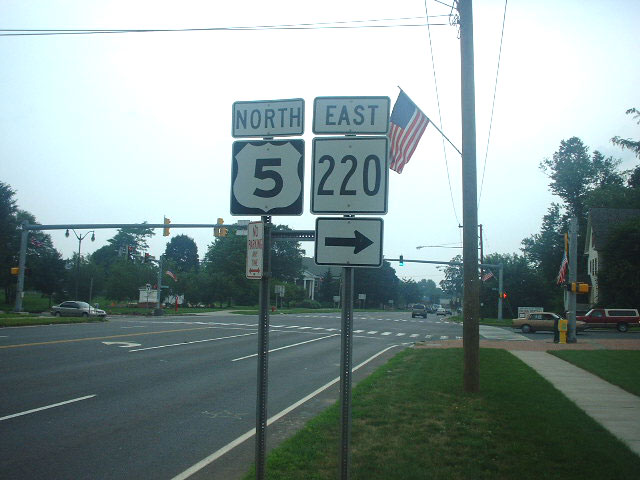In this outdoor photograph, the central focus is a pair of street signs prominently positioned against a backdrop of a city intersection. The left signpost displays two stacked signs: the top sign is a black and white rectangle indicating 'North', while the square sign below it features the number '5'. Adjacent to this, on the right signpost, the upper sign is a white rectangle with 'East' written in black, and the square sign below it bears the number '220' in black on a white background. Additionally, a rectangular sign positioned beneath this indicates direction with a black arrow pointing to the right on a white background. 

On the original left signpost, there is also a white and red 'No Parking' sign. Behind these street signs, the image captures an intersection, with visible roads suggesting a city or town setting. A prominent wooden pole stands out, equipped with power lines and adorned with a vibrant red, white, and blue American flag. The background is crowned by a sky interspersed with patches of blue and scattered white clouds, adding a natural element to the urban scene.